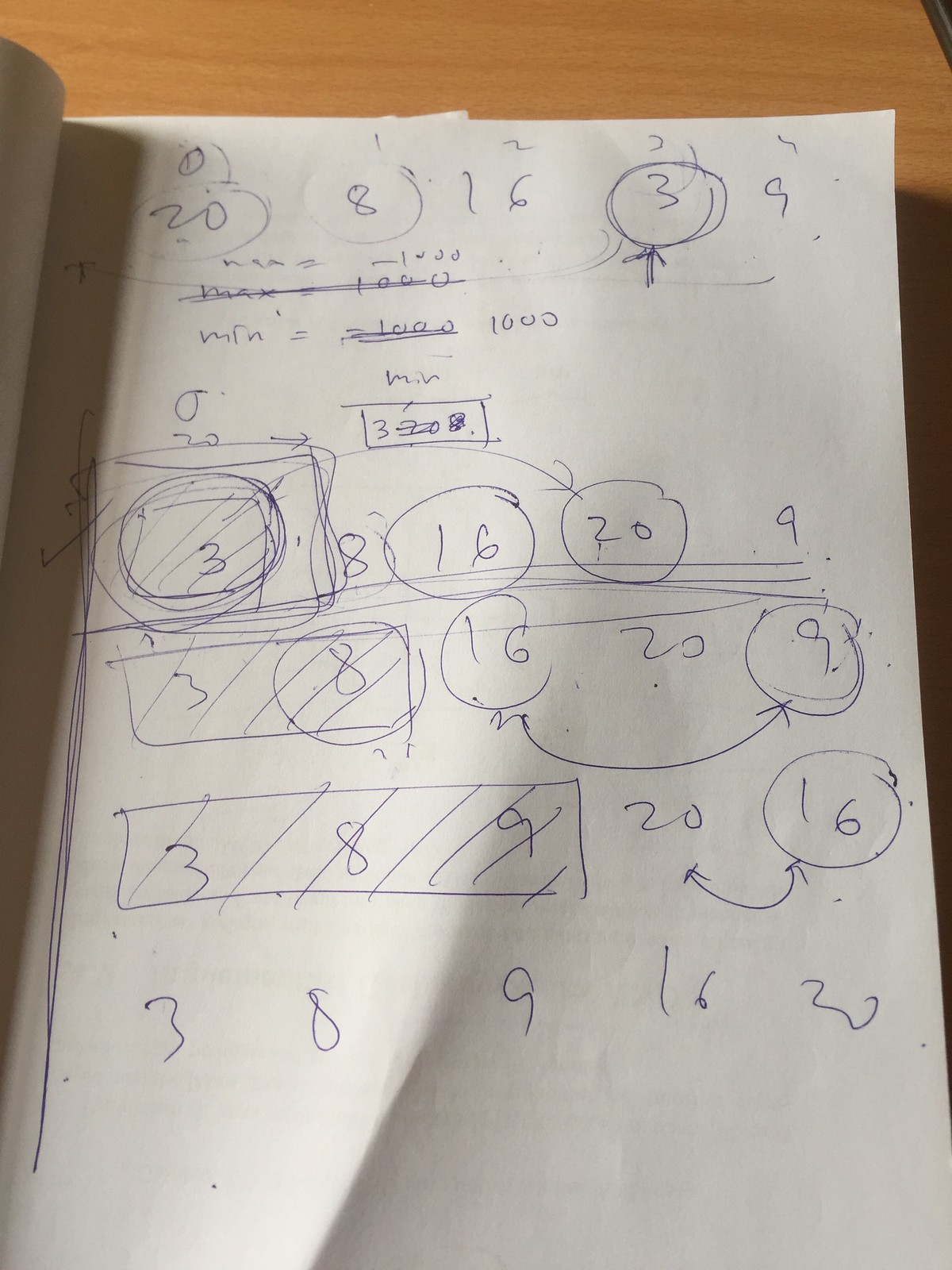Caption: 

A detailed image of a wrinkled and folded piece of paper placed on a brown table. The surface of the table forms the background, with shadows cast on both the left-hand and right-hand sides of the scene. The paper contains various numerical entries and drawn shapes in a somewhat chaotic layout. 

At the top center of the paper, a sequence of numbers is noted: 0, 20, 8, 16, 3, 9, 4. Toward the bottom left of the paper, there are scratch marks adjacent to the notation "Min equals 1,000." Below this note, on the left, another sequence reads "0, 20." To the right of this entry, the word "min" is written. A square near this section contains the numbers "3, 2, 0, 8."

Further details include a circle drawn on the side with a square enclosing the number "3," alongside scratches indicating "8." Moving horizontally from left to right, the numbers 16, 20, and 9 are listed, with additional scratch marks underneath. To the left, a rectangle enclosing the numbers "3" and "8" is next to a circle containing the number "8." Beyond this, 16 and 20 are written without any enclosing shapes, followed by the number 9.

A line arrow connects the number 16 to the number 9. Another rectangle, scratched out, holds the numbers 3 and 9 inside it. Further to the right, the number 20 appears again, followed by 16. An arrow connects the two sets of 20 and 16.

At the very bottom of the paper, the numbers are listed in a sequence starting from 1 on the left, followed by 3, 0, 9, 16, and 20 in the bottom row.